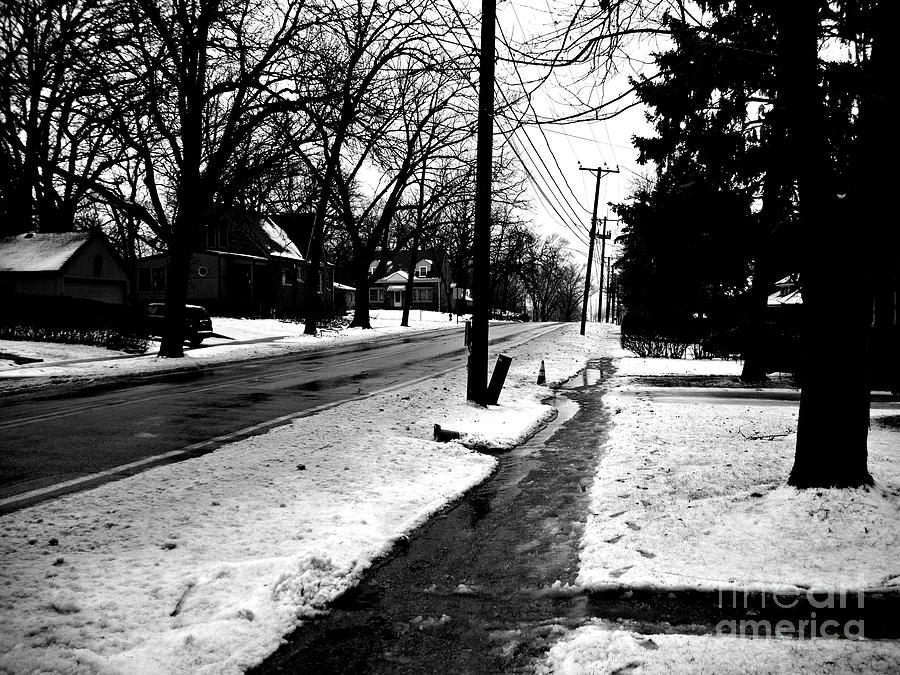The image is a square, black-and-white photograph of a suburban neighborhood taken during the winter daytime, with a cloudy sky overhead. The scene is devoid of people and activity, focusing instead on the quiet, snow-blanketed landscape. At the center, a two-lane road has been cleared of snow but remains wet and slushy, hinting at recent snowfall. The sidewalk parallel to the road is similarly cleared but appears icy. Power lines run along wooden telephone poles that line the sidewalk. To the left, bare-branched trees and typical suburban homes with boxy shapes and triangular roofs dominate the scene. The lawns are covered in thick snow, marred only by footprints. To the right, a mix of bare trees and a couple of leafy pine trees frame additional houses. One house has an SUV parked in its driveway—the only apparent vehicle in the image. A barely legible watermark in the lower right corner reads "The Art America." This serene winter scene captures the quiet and stillness of a suburban neighborhood blanketed in snow.